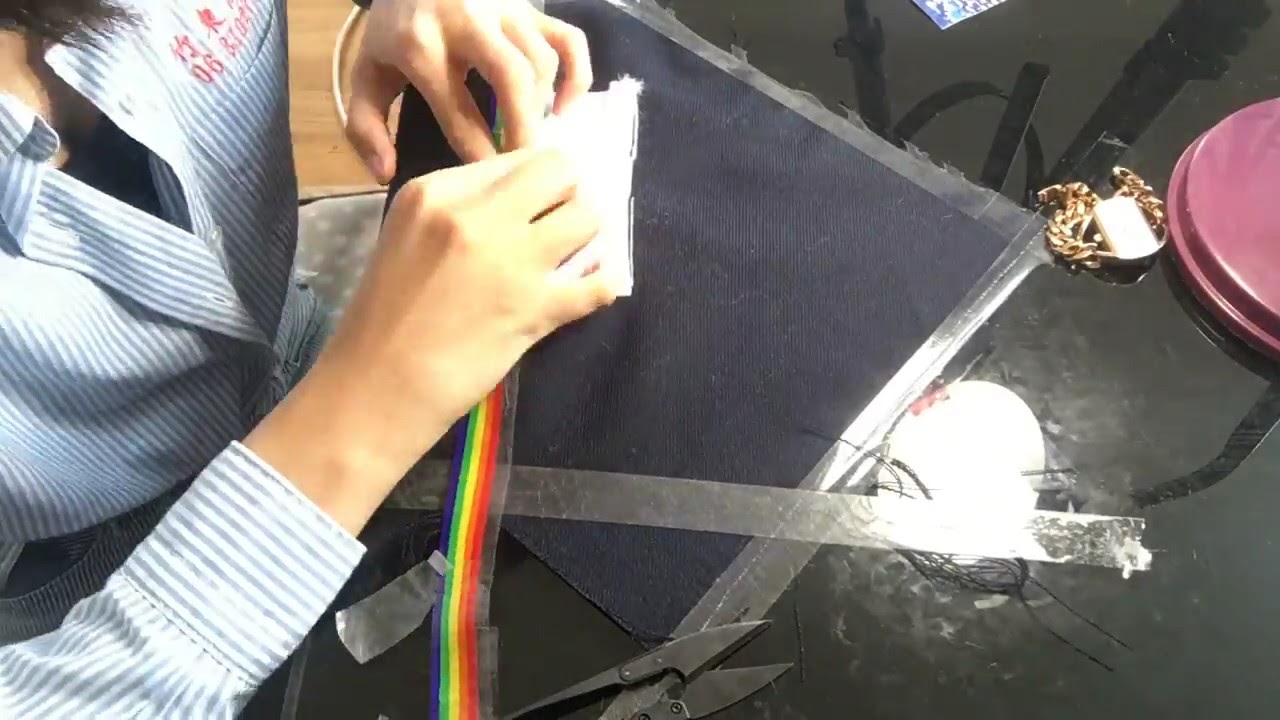The image captures a scene where a woman, identifiable by her hands and black hair, is diligently working on a project at a reflective surface. She is dressed in a blue and white striped button-up shirt with the shirt's numbers "06810" and possibly Chinese or Japanese characters inscribed above them, partially visible. She appears to be wearing a black tank top underneath the shirt. The table she is working on holds various items including scissors, black and clear tape, threads, a rainbow-colored ribbon, a bracelet-like object, and a pink circular item which might be a light base. She is laying a rainbow-striped ribbon onto a piece of dark fabric, securing it with tape. The fabric appears to be around a foot in diameter, possibly rectangular, with the black material also fastened with tape. The overall atmosphere suggests she is either repairing or creating something from scratch, meticulously aligning the pieces with care.